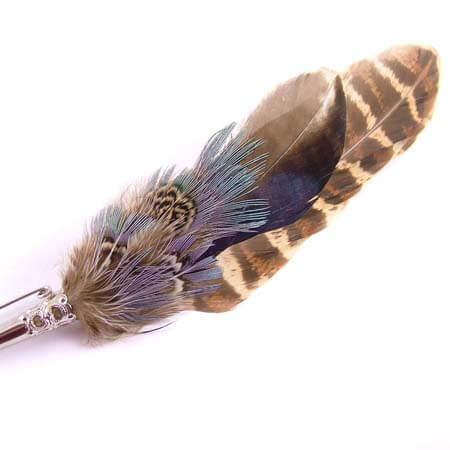The image showcases a collection of various feathers arranged on a white background, likely attached to a writing instrument or crystal holder that extends from the bottom left to the top right. In the very back, a large, illuminated feather exhibits dark brown, light brown, and white stripes. Positioned in front of it is another feather featuring a stark dichotomy: it's almost black on one side and light brown on the other. Below and in front of these larger feathers are smaller ones with a bluish hue and a subtle striped pattern at the base. Some of the smaller feathers have elongated, eyelash-like filaments. Towards the top, the feathers become denser, exhibiting a blend of blue, purple, and brownish tones, along with fine, thread-like details. The arrangement likely suggests a feather pen, with the intricate, variegated feathers adding texture and depth to the overall composition.